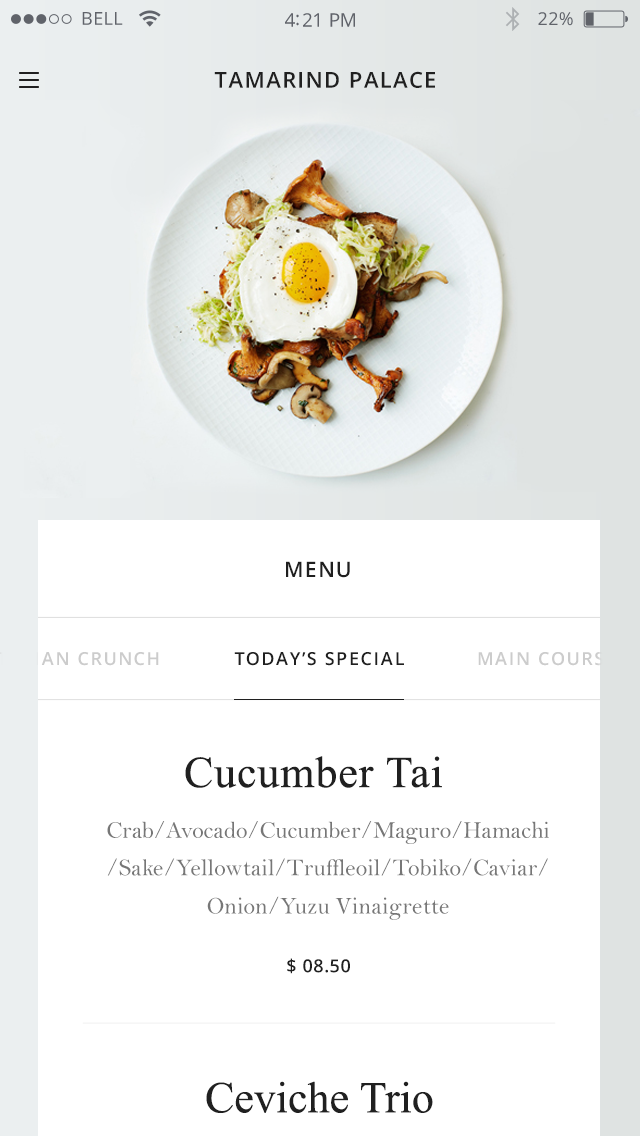The image is a vertical rectangular photograph, likely taken from a cell phone. At the very top center of the image, the screen displays the current time as "4:21 PM" in white font, along with a battery indicator on the right side showing 22% remaining, with the battery icon appearing mostly empty.

In the upper left corner, there are three horizontal black lines, commonly representing a menu or navigation icon. The focus then shifts to the middle of the image where the name of a restaurant is displayed prominently: "TamarinD Palace."

Directly below the restaurant name, there is a circular white plate viewed from above. This plate features a sunny side up egg on top, garnished with mushrooms, lettuce, and other ingredients. The plate is set against an off-white background.

Further down on the image, still on the off-white background, there is a vertical white section that contains the word "Menu" written in black lettering at the top. Below "Menu," in light gray writing, is the word "Crunch." The next section, written in black font with an underline, states "Today's Special." To the right of this, in gray font, it reads "Main Course."

Underneath the heading "Today's Special," in bold black font, the item "Cucumber Thai" is listed. Below this, in regular black font, the details of the dish are provided: "Crab / Avocado / Cucumber / Maguro / Hamachi / Saki / Yellowtail / Truffle Oil / Tobiko / Caviar / Onion / Yuzu Vinaigrette." The price for this dish, boldly listed, is "$08.50."

Following this, the next menu item, "Ceviche Trio," is also displayed in bold black font, indicating it is another special of the day.